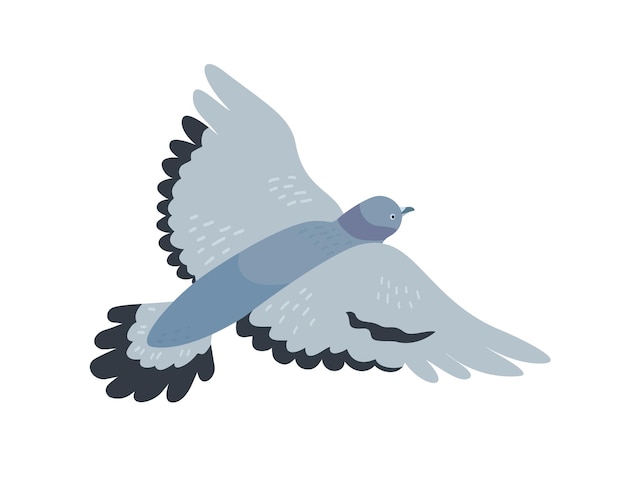The image depicts a piece of clip art featuring a light blue-gray bird flying diagonally towards the upper right. The bird’s wingspan is prominently showcased, with the wings being primarily light blue but featuring dark blue tips and a wavy dark blue line on the right wing. Its tail feathers mirror this coloration, light blue with dark blue tips. The bird's body is capsule-shaped and of a slightly deeper blue-gray shade, with a subtle purplish stripe around the neck area. It has a distinct white eye with a black pupil and a beak that transitions from white near the base to blue at the end. The style is reminiscent of basic, simple Microsoft clip art, combining shades of light and dark blue with gray undertones for a cohesive yet detailed appearance.